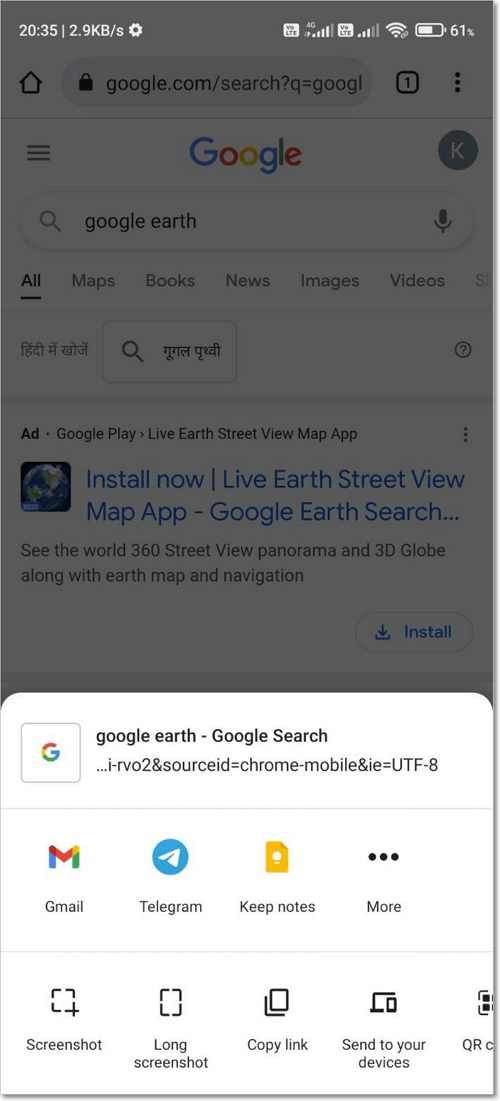This is a detailed screenshot of a smartphone's display captured at 20:35. The top status bar reveals a data transfer rate of 2.9 kb/s next to the settings icon. There are two internet connectivity icons, and the battery is at 61%. The background showcases a Google search bar with the truncated URL "google.com/search?q=G O O G L...". Beneath the search bar, the Google logo is prominently displayed, with each letter in its respective color: blue 'G', red 'O', yellow 'O', blue 'G', green 'L', and red 'E'. To the right, a dark gray circle encloses the letter 'K'. 

Below the search bar, "Google Earth" is typed in, leading to a navigation bar with categories such as All (highlighted), Maps, Books, News, Images, Videos, and More. The search results display Chinese characters, suggesting the use of non-English search terms. An advertisement follows: "Google Play, Live Earth, Street View, Map, App" with an Earth icon and a call-to-action "Install now." Detailed text promoting these apps describes features like "See the world 360, Street View, Panorama, and 3D globe along with Earth, Map, and Navigation."

In the foreground, a white overlay partially obscures the content. This overlay features a Google-branded box with a 'G' symbol, indicating "Google Earth, Google Search," followed by a long URL ending in UTF-8. At the bottom, four app icons are visible: Gmail, Telegram, Keep Notes, and a fourth option for more apps denoted by an ellipsis. Finally, options for actions include "Screenshot," "Long screenshot," "Copy link," "Send to your devices," and a partially visible choice starting with "QR."